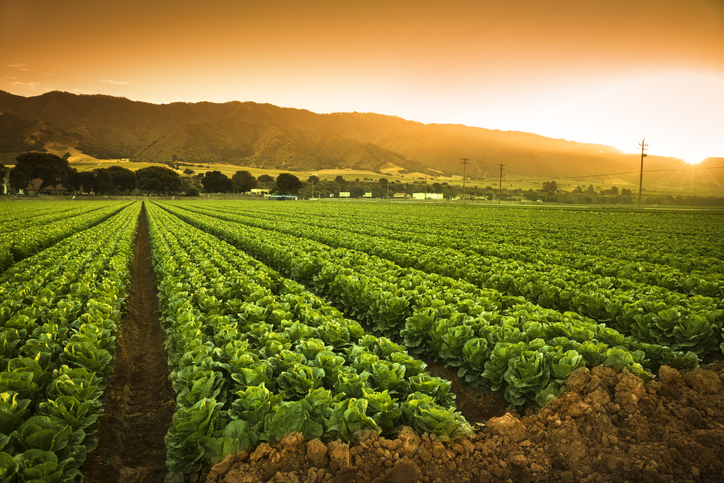The photograph depicts an expansive farm field meticulously planted with rows of green lettuce stretching into the distance. The well-ordered lines of lettuce are separated by turned-up brown soil, creating a rhythmic pattern that draws the eye toward the horizon. In the immediate foreground, freshly tilled earth defines the boundary of the cultivated area. As the field extends backward, it meets a row of trees that lines the edge, beyond which there are subtle indications of a road suggested by scattered signs. Rising from the valley behind the trees are large, tree-covered hills that recede into the distance, bathed in the warm hues of a rising or setting sun. To the right of the image, a series of power poles march in parallel with the lettuce rows, guiding the observer's gaze towards the distant houses nestled at the base of the hills. This harmonious blend of agricultural dedication and natural beauty is accentuated by the first light of dawn or the last light of dusk, casting a serene glow over the entire scene.